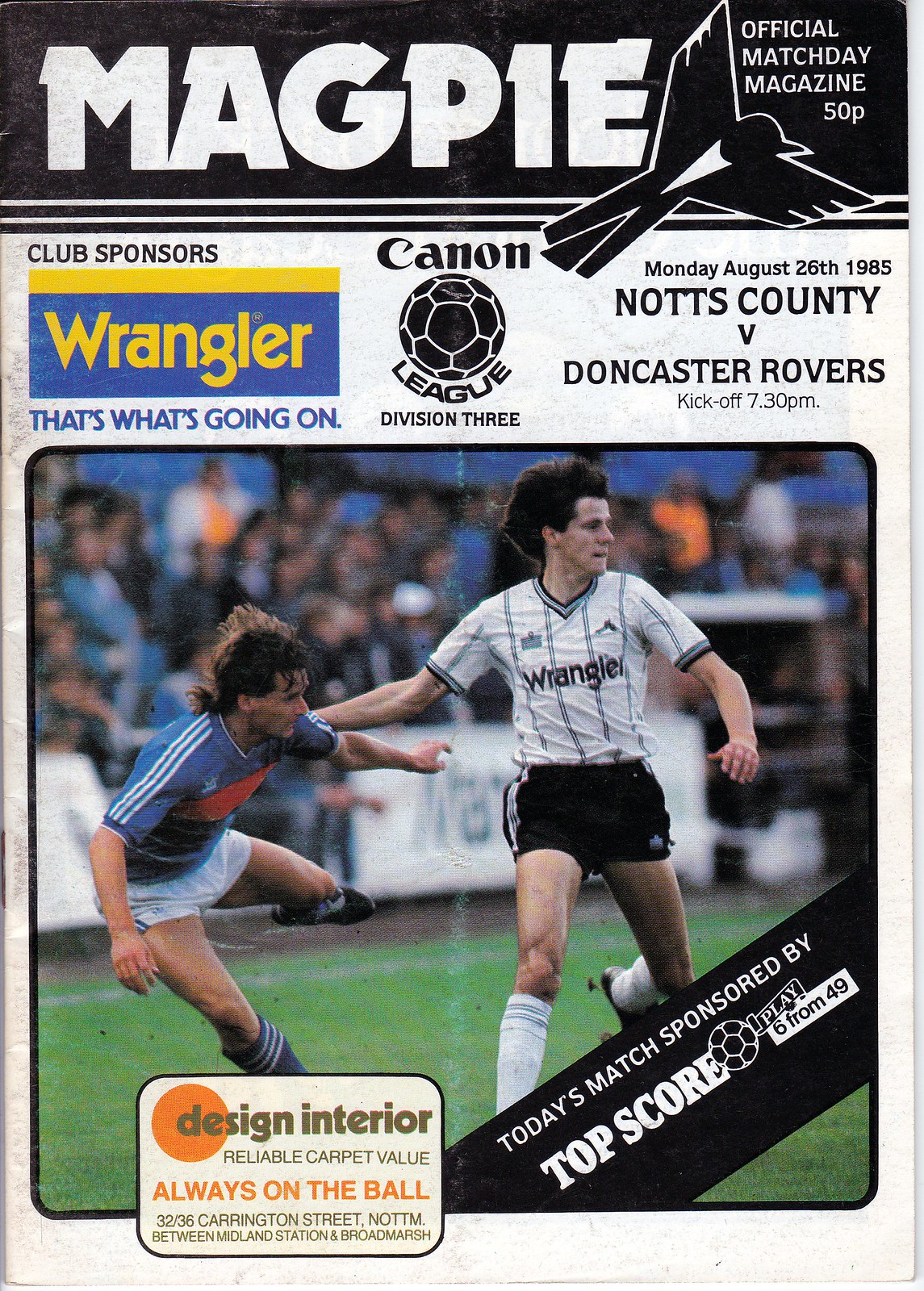This is the cover of the official Match Day magazine, titled "Magpie," priced at 50p. The cover prominently features a large color photograph of two opposing soccer players in action. One player, dressed in a blue jersey with white shorts, has his leg up, appearing as if he is about to fall. The other player, clad in a white v-neck jersey with vertical gray stripes and black shorts, stands upright. The blue jersey bears the word "Wrangler," similar to the style of the famous jean company.

A black banner stretches across the top with the magazine's title "Magpie" in bold white text next to an illustration of a magpie bird. Directly beneath this banner, it lists the club sponsors, Wrangler and Canon, with the Canon League Division Three logo. It notes the match specifics: "Monday, August 26, 1985, Knotts County vs. Doncaster Rovers, kickoff at 7:30 p.m."

On the lower right corner of the photograph, a black diagonal ribbon reads, "Today's match sponsored by Topscore, play 6 from 49" in white text, accompanied by an icon of a soccer ball. Additionally, the bottom left corner contains an inset advertisement for "Design Interior, Reliable Carpet Value," with the tagline "Always on the Ball."